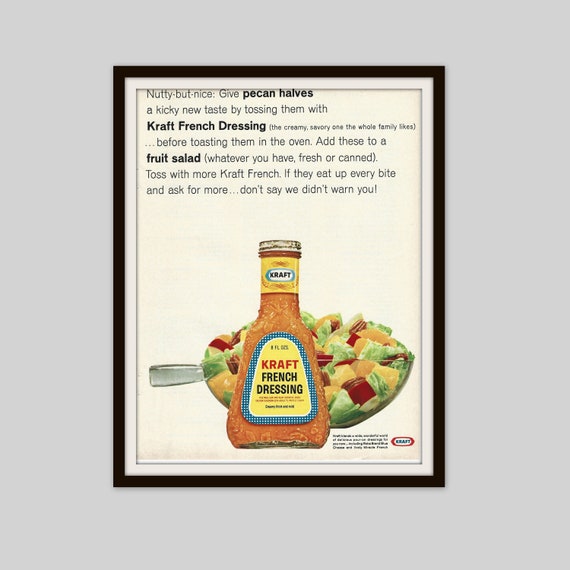This detailed caption combines the repeated and critical elements from each speech:

The framed advertisement, mounted on a gray background wall, features a vintage Kraft French dressing bottle, likely from the 1960s or 70s. The black metal frame surrounds a thin matting that highlights a white backdrop, showcasing the iconic tapered glass bottle filled with orange dressing. The bottle has a rounded top and a distinctive label with blue check patterns, a yellow center, and text reading "Kraft" in red and "French Dressing" in black. Behind the bottle, a bowl of salad filled with vibrant red, yellow, and green vegetables, pecans, and possibly chunks of apple. The bowl, which is clear glass with a handle on the left, adds depth to the nostalgic scene. At the top of the advertisement, the text reads, "Nutty but Nice. Give pecan halves a kicky new taste by tossing them with Kraft French Dressing, the creamy, savory one the whole family likes. Before toasting them in the oven, add these to a fruit salad, fresh or canned. If they eat up every bite and ask for more, don't say we didn't warn you." This classic ad, preserved in a frame, exudes charm and culinary nostalgia.